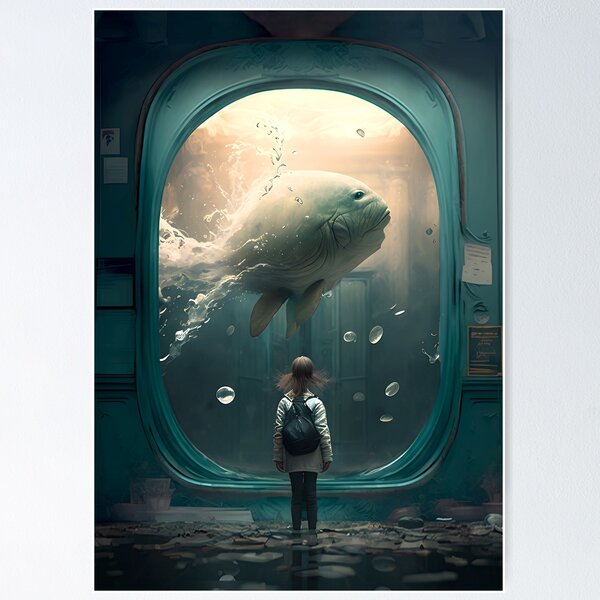A digitally created image likely produced through Photoshop or AI generation features a young girl standing with her back to us, fixated on a massive fish within an aquarium window. She wears a white or light grey hoodie, a blue backpack, and black pants or leggings. A breeze appears to have lifted her hair up into the air, adding a sense of dynamic movement to the scene. The girl stands on a dark, possibly black tiled ground which has scattered debris. She is surrounded by dim indoor lighting, yet the aquarium tank glows with light possibly from above, highlighting the scene dramatically. The main focal point is the enormous fish, about three times the size of the girl, swimming energetically and creating splashes and bubbles. Although we can’t see her face, her body language suggests she is awestruck by the sight. In addition to the visual elements, there are two tiny unreadable signs on either side of the viewing window. The overall atmosphere is one of wonder and amazement, capturing the girl's mesmerized state.